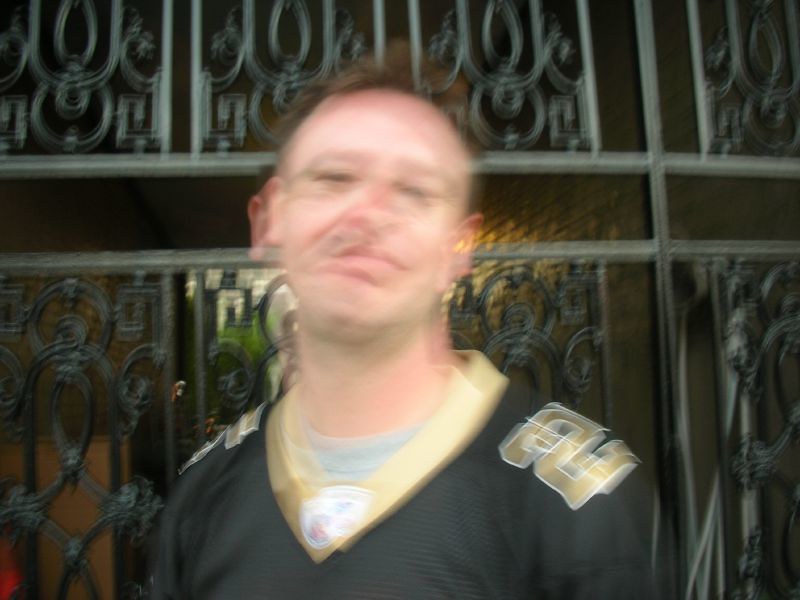The photograph features a white male standing outside a decorative, wrought iron black gate. The image is notably blurry, suggesting either the subject or the camera was in motion during the capture, resulting in a double image effect particularly noticeable around the man's face. He has short to medium brown hair which is receding and shaved on the sides, giving him a balding appearance. His facial expression is neutral to slightly sad, with his eyes squinted and a faint smile. The man is dressed in a black New Orleans Saints NFL football jersey, distinguished by a gold collar featuring a white emblem at the center and the number two on the shoulder. Under the jersey, he wears a silver-gray undershirt. Behind him, the ornate gate is detailed with long, stick-like shapes and oval designs, and it appears to frame a tunnel or passageway in the background.